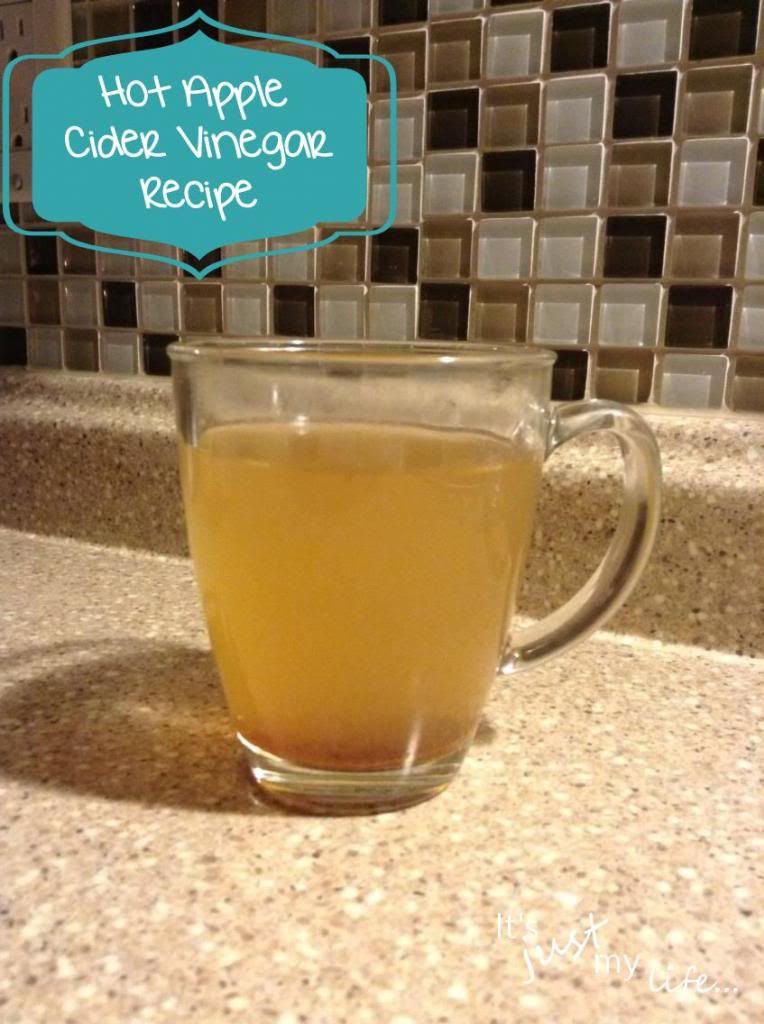The image depicts a close-up of a clear glass mug containing a light orange liquid, likely hot apple cider vinegar, as suggested by the text in the top left corner. The mug, complete with a handle, sits on a countertop that appears to be either low-quality granite or a textured material resembling it, featuring blue, white, and black specks. Additionally, the countertop might be marble or plastic. The background showcases a kitchen wall adorned with small, randomly arranged ceramic tiles in shades of white, black, gray, and tan. Overlaying the image is a Photobucket watermark, characterized by the site's logo—a set of concentric circles mimicking a camera lens. Below the logo, a white banner with the tagline "Protect more of your memories for less!" further confirms the image's stock photo nature.